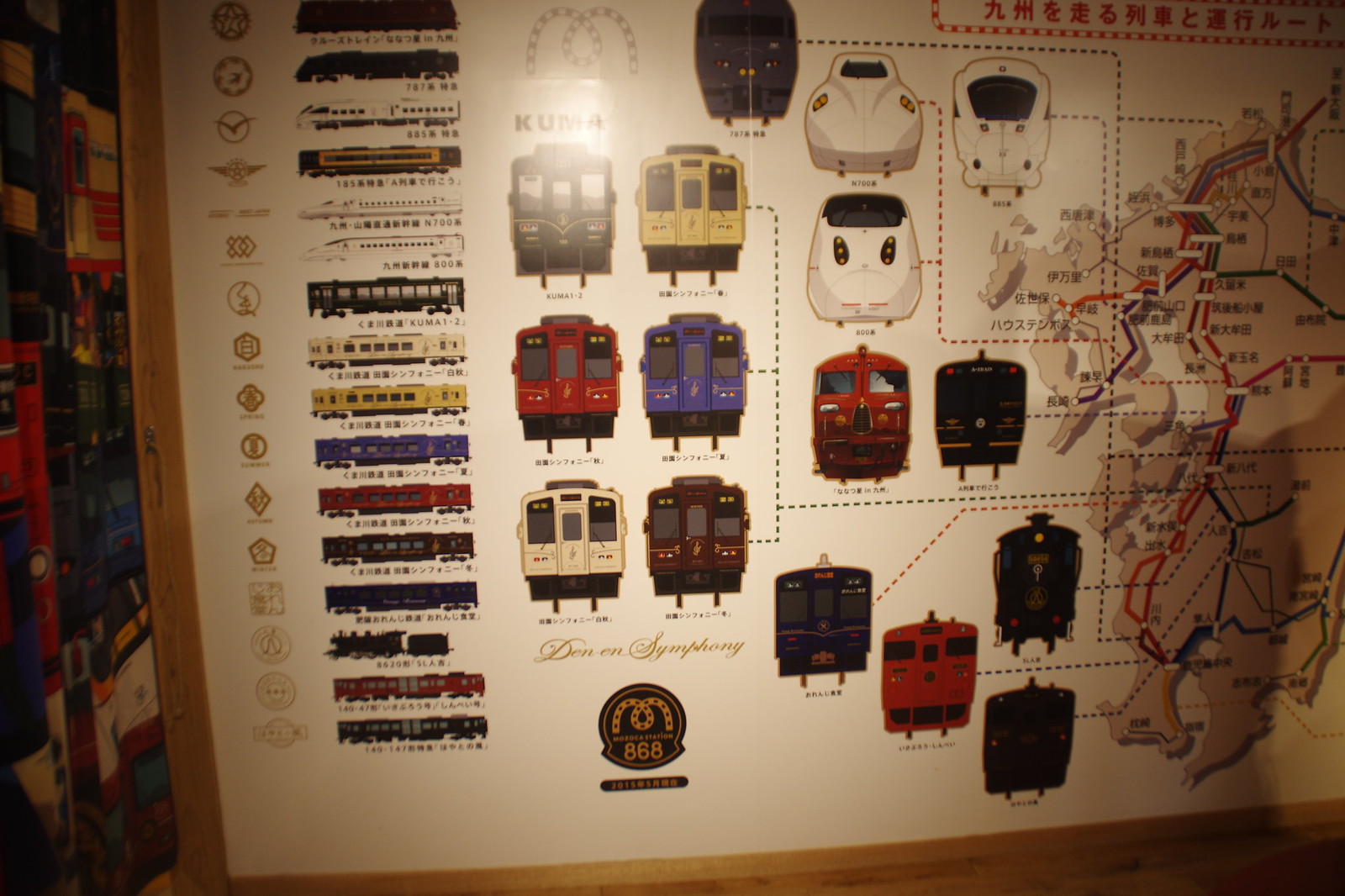The image depicts an informational display board, likely situated in a museum or similar venue, showcasing various trains used in Japan. The display is bordered by wooden edges and features a white background filled with detailed information written in kanji, which includes pronunciations, route names, and town names. Centrally placed on the board are images of 16 different trains, each labeled and accompanied by their corresponding brand icons. The display provides a comprehensive overview of the trains' routes and the locations they serve, including the Shinkansen and other colorfully depicted trains. The top right corner of the board contains additional Asian lettering, enhancing the informative nature of the exhibit.